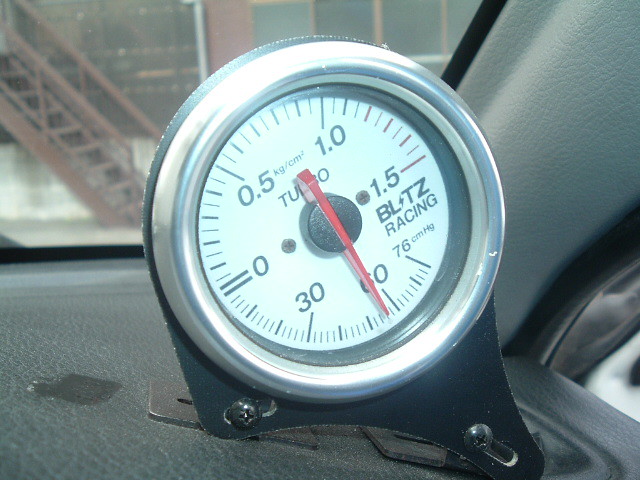A close-up image displays a gauge mounted on the dashboard, likely on the passenger side, of a car with a black interior. The gauge is housed in a glossy, black plastic casing with a curved window, providing a view from both the front and the side. Its scale is numbered with unusual increments: starting from 60 at the bottom, moving leftwards to 30, then to 0.5, 1, and finally 1.5 beyond the midpoint. The gauge itself reads at 0.7 kg/cm², a unit likely indicating pressure. Prominently featured on the gauge is the branding "Blitz Racing." Outside the car, the scene includes a building with a large window, a brown storefront, and a distinctive brown staircase leading upwards to the left.